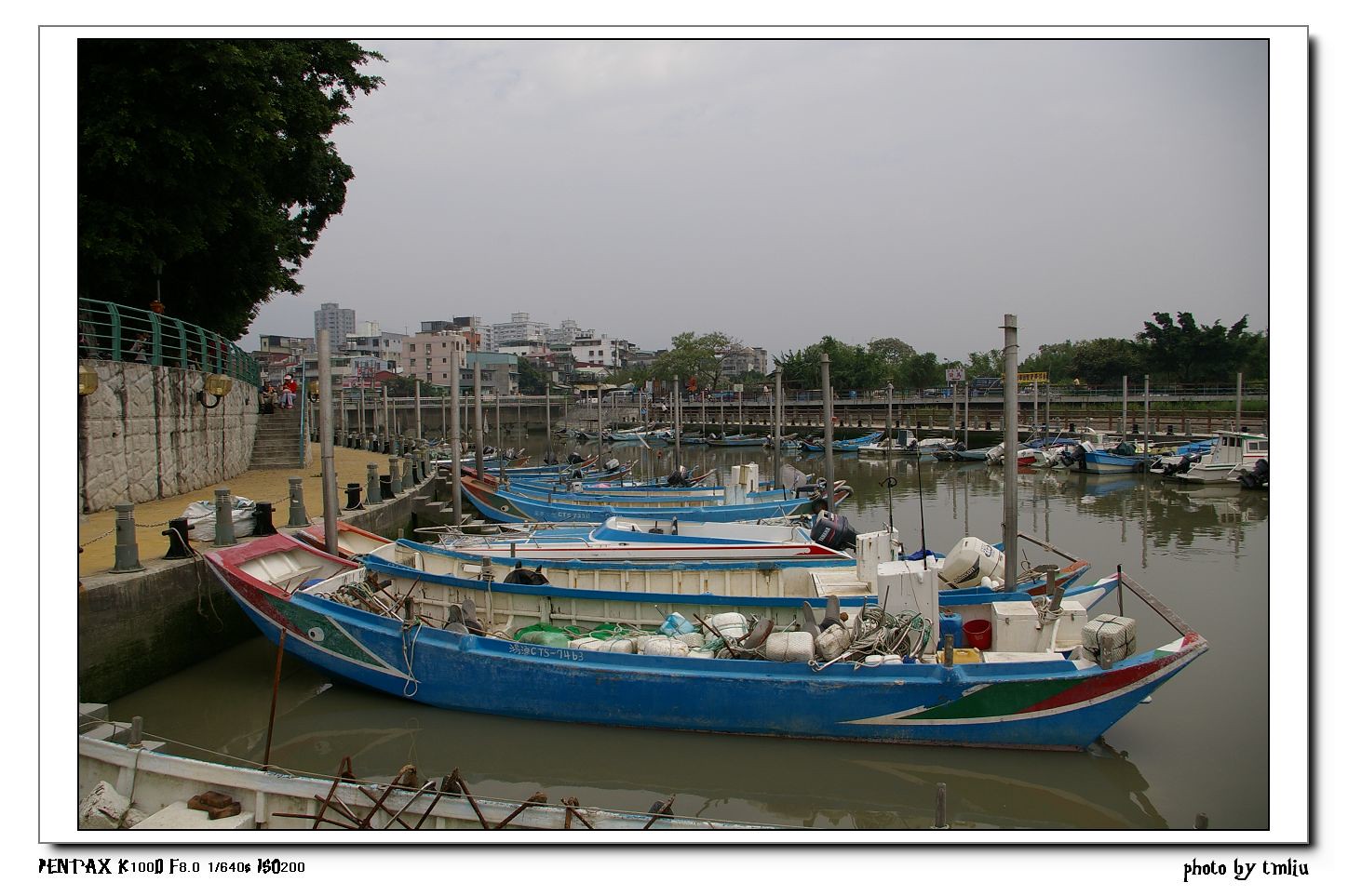This wide, horizontal color photograph, labeled "Photo by TMLIU" and shot with a Penpax K1000 at 200 ISO, captures a picturesque marina scene. The image, set against a white background with a black shadow beneath, features a bustling boat dock along a river or canal. Several long, low boats, primarily painted in shades of blue with green, red, and white accents, are roped to a curved stone promenade. This walkway, equipped with bollards for securing the boats and topped by a green iron fence, offers staircases leading up from it. Among the boats, some appear to be passenger vessels with benches, while others seem designed for fishing, all fitted with motors at the back and devoid of sails. The marina is bustling with moored personal boats, and the scene is framed by large trees sprouting from the retaining wall adjacent to the promenade. In the distance, additional docks and boats can be seen, alongside the silhouette of city buildings under a cloudy sky.